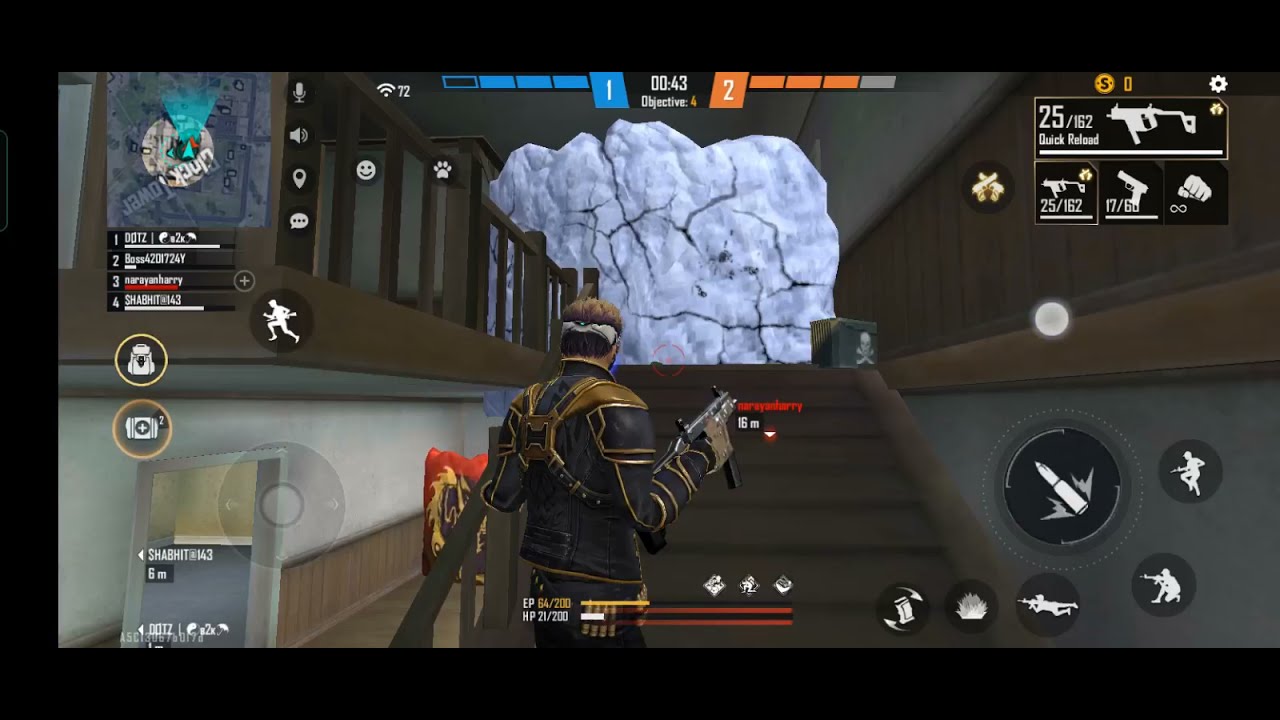In this video game screenshot, we see a character facing away from the camera, standing at the base of a wooden staircase. He is clad in a futuristic black outfit with gold detailing along the sleeves and bottom, featuring an unusual combination of silver-plated armor and what appears to be jean material instead of traditional leather. The character also sports a headband, potentially goggles, and brown gloves, with a rifle securely held in his right hand. A gold-colored sling crosses over his black jacket, and there’s a case on his hip that likely contains extra ammunition. The setting appears to be inside a home, characterized by hardwood floors and paneled walls, transitioning to white walls and ceiling above. At the top of the stairs, there is a large white stone with black veining, and to the left, a balcony can be seen. Additionally, a large grayish rock and big red pillow with gold markings are visible in the background. The game interface includes various icons and text, with a "quick reload" indicator on the right side and a mini-map in the top left corner.